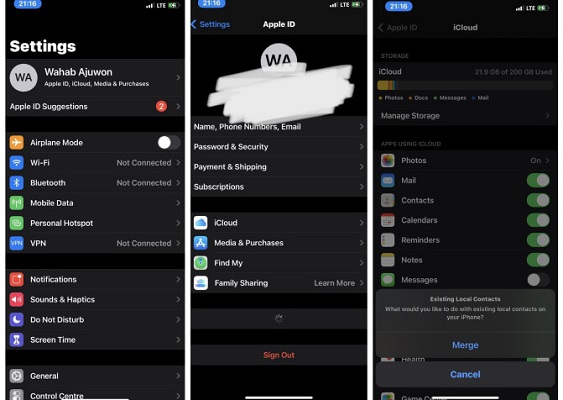Three side-by-side screenshots of a smartphone settings app are displayed against a black background with white text. 

- The first screenshot showcases the main Settings menu, revealing options such as "Settings," "Wahab," "Ojuwon," and "Apple ID Suggestions." Below these are toggles and sections for "Airplane Mode" (off), "Wi-Fi" (not connected), "Bluetooth" (not connected), "Mobile Data," "Personal Hotspot," and "VPN" (not connected). Further down, it lists categories for "Notifications," "Sounds & Haptics," "Do Not Disturb," "Screen Time," "General," and "Control Center."

- The middle screenshot delves into the Apple ID settings. Here, "Settings" and "Apple ID" are visible at the top, followed by standard icons. Notably, a section labeled "WA" features heavy white scribbling to obscure part of the information. The visible options include "Name, Phone Numbers, Email," "Password & Security," "Payment & Shipping," "Subscriptions," "iCloud," "Media & Purchases," "Find My," "Family Sharing," and "Learn More." Additionally, a loading indicator appears near "Sign Out."

- The third screenshot pertains to iCloud settings, detailing the management and storage options. It lists the following options: "Photos" (on), "Mail" (yes), "Contacts" (yes), "Calendars" (yes), "Reminders" (yes), "Notes" (yes), and "Messages" (no). It also includes actions for "Existing Local Contacts" to "Manage or Merge," followed by a "Cancel" button.

Each screenshot provides a snapshot of various functional settings within the phone, presented with clarity against the chic and sleek black background.